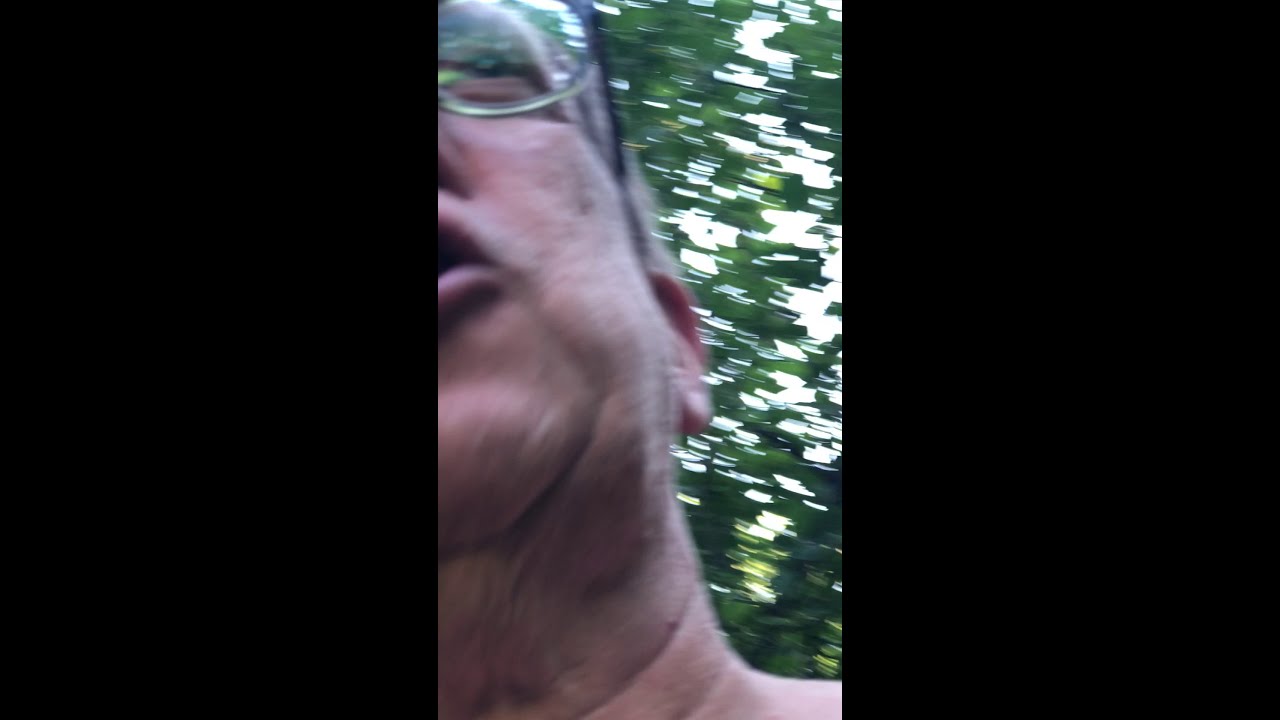The image is a portrait-oriented photo featuring a close-up shot of an older Caucasian man, possibly in his early 60s, captured from a low angle. The photo composition has black borders on the left and right, making the center strip narrow and tall. His face is only partially visible, highlighting the underside of his chin, neck, and the right side of his face. He is wearing glasses with black upper rims and frameless bottoms. His mouth is open, suggesting he's mid-conversation, possibly on a video call like FaceTime. The image background shows streaks of green and white, resembling trees and the sky, indicating he is outside. His neck displays deep wrinkles and he has a double chin, with hints of a gray mustache and gray hair visible.